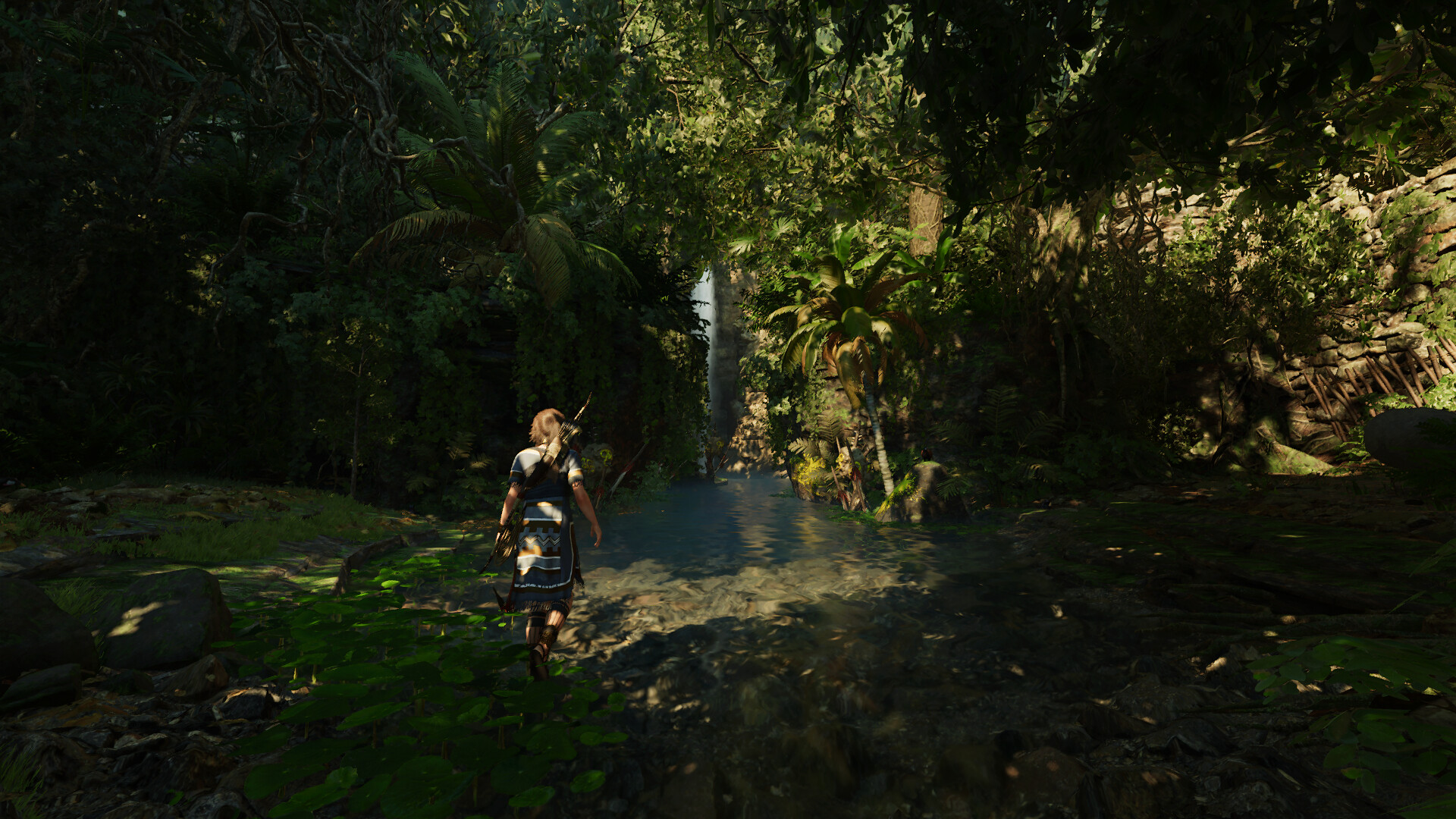In this detailed in-game screenshot, we see a dense, tropical jungle environment characterized by thick clusters of trees, shrubs, and a variety of vibrant green foliage, including large palm leaves and some plants with neon green and dark emerald green hues. The scene is dominated by an expanse of water positioned centrally, with additional water features extending toward the right-hand side, hinting at a waterfall. Large gray stones, moss, green grass, and algae populate the bottom left corner. A video game character stands with their back to the viewer, walking toward the water. They sport a blue and white outfit, brown hair, boots, and a kilt. Strapped to their back is a weapon that resembles either a bow and arrow or a sword. Sunlight filters through the dense jungle canopy, illuminating the scene and adding to the rich, immersive atmosphere of the game.